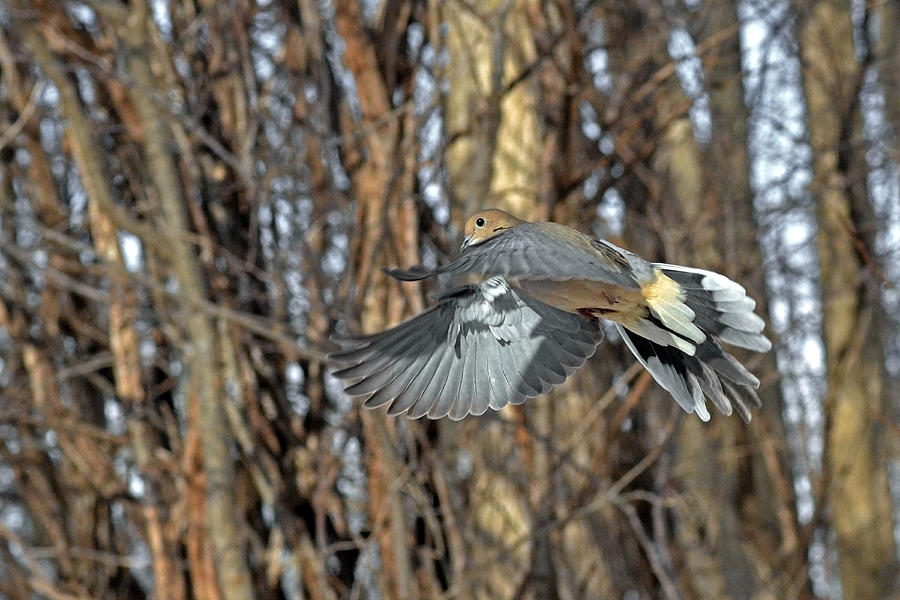In this detailed photograph, taken in a wintery, leafless wooded area, a bird, likely a mourning dove, is captured in mid-flight against a backdrop of various bare trees and a light blue sky. The bird is the central focus, with its wings extended forward as if preparing for the next thrust. The bird's body displays a cream to beige coloration, while its wings and tail feathers are predominantly dark gray with lighter gray, almost white tips. The head of the bird is a brownish-gray color with a distinctive black beady eye. Its legs are tucked up close to the body, reminiscent of an airplane's landing gear. Subtle sunlight filters through the scene, adding a gentle glow. Overall, the image beautifully encapsulates the serene, still moment of the bird's flight amidst the stark, wintery backdrop.